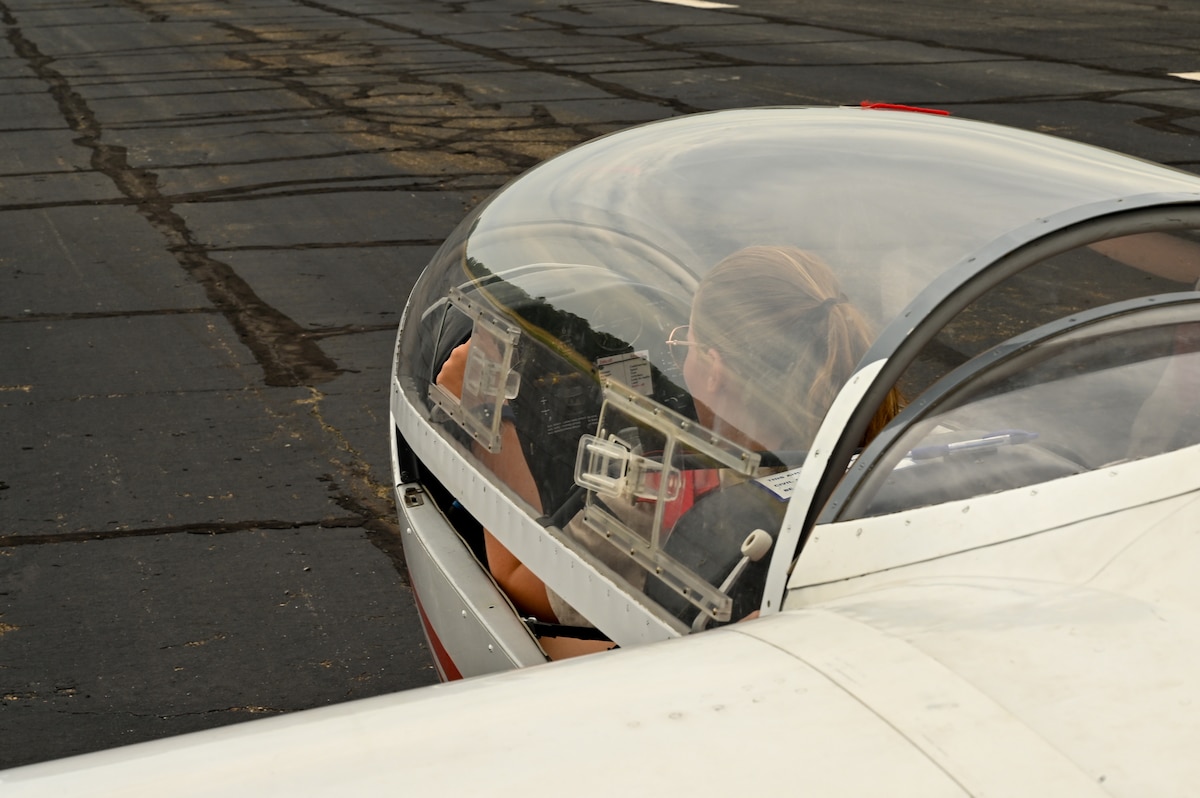In this detailed image, a dirty blonde-haired woman, wearing silver-rimmed aviator sunglasses, is seated in the cockpit of an ultralight plane. She's inside a plexiglass canopy that frames her against a rugged runway. She's dressed in a short-sleeve gray shirt and has her hair pulled back into a ponytail. 

Her hands are active: one appears to be reaching up towards a small square window on the side of the bubble-like canopy, and the other might be on the throttle. The cockpit, seemingly a two-seater though unoccupied, has gray paneling in front of her and straps securing her in place.

Behind her head is the white wing of the ultralight, where bolts are visible at the junction with the glass canopy. Below her forearm, towards her elbow, there is a noticeable opening. In the background, the beat-up black tarmac is marked with various tar repairs and faded lines, indicating a less-maintained airstrip. Slightly visible plates and bolts around the area suggest detailed structural features of the white plane, which also sports a red stripe on the bottom of the fuselage near the nose. The woman appears poised for takeoff, with the propeller likely mounted at the rear of the craft.